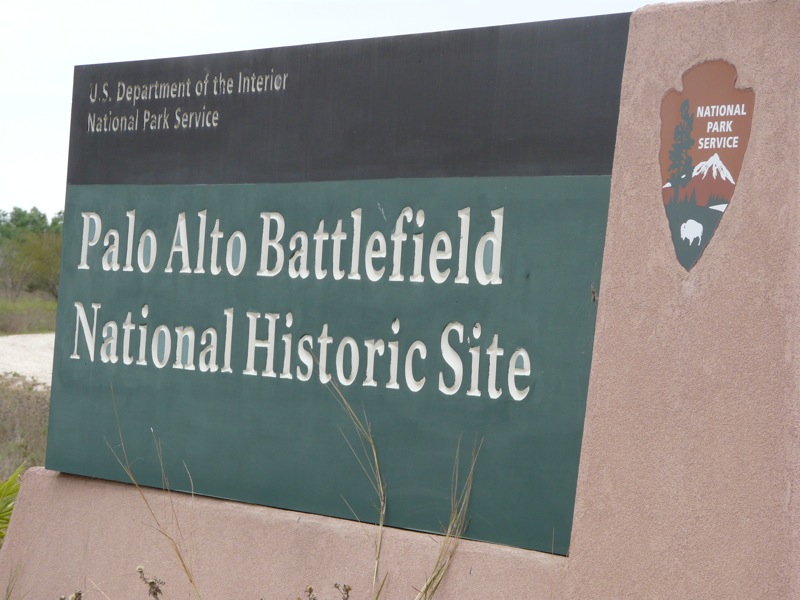This photograph captures a weathered, official sign at the Palo Alto Battlefield National Historic Site, maintained by the U.S. Department of the Interior National Park Service. The sign is centrally positioned in the image, made from a long concrete structure with varied textures and colors. 

At the top left, in black, bold text, it reads "U.S. Department of the Interior National Park Service." Positioned centrally below, in green with white lettering, is "Palo Alto Battlefield National Historic Site." To the right, carved into the concrete, is the National Park Service badge featuring trees, mountains, and a bison, rendered in a palette of black, white, and a distinctive brownish red.

The scene includes a mix of colors: black, greenish-gray, white, red, and a brownish-pink hue from the concrete. The overcast sky adds a solemn, serious tone to the setting. Surrounding plants and foliage, some appearing to grow up into the sign, emphasize the natural environment and the historic context of the site. Visible green leaves and branches hint at a wooded area to the left side of the frame, enriching the natural backdrop.